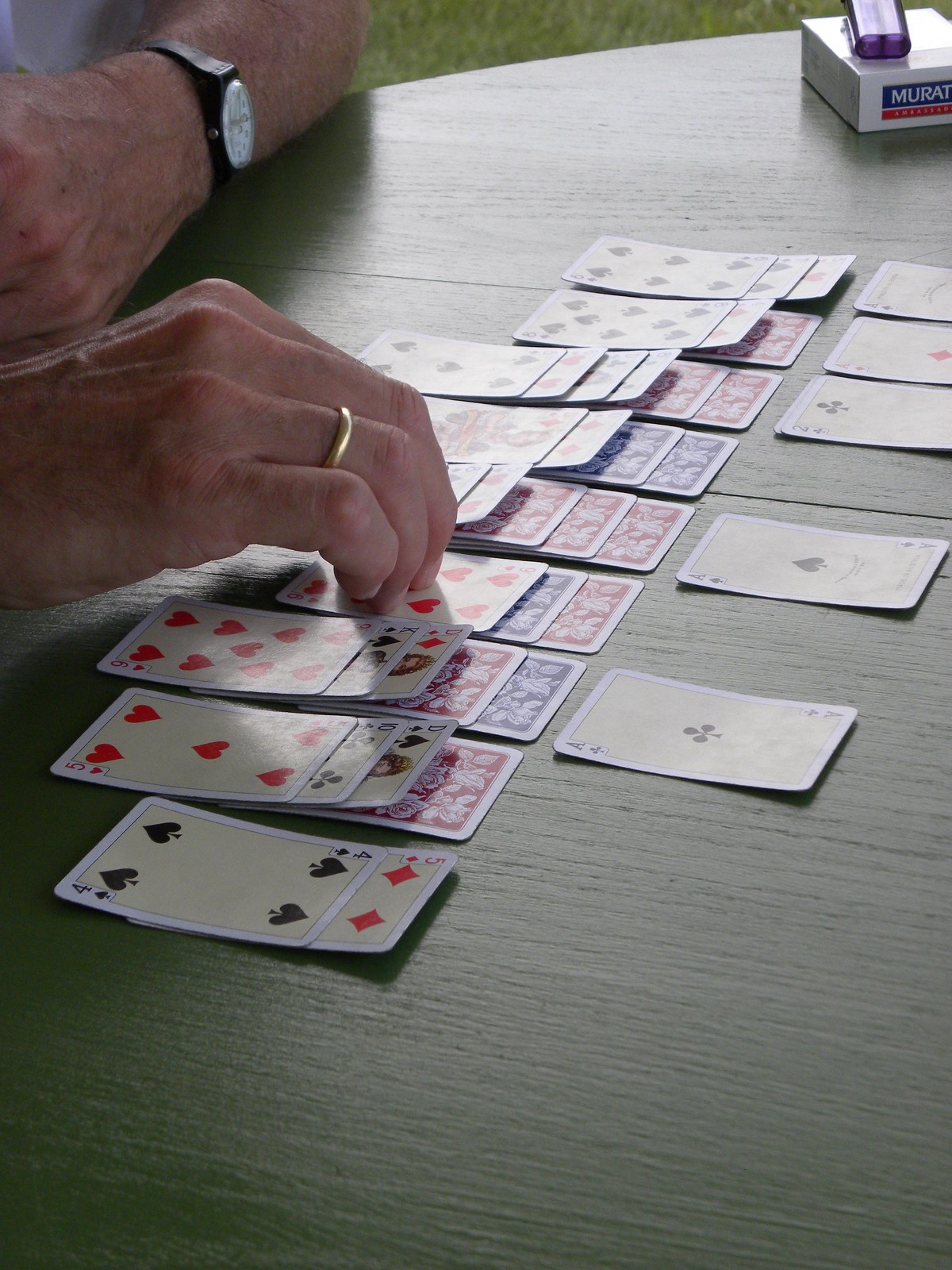The color photograph captures a close-up view of a dark green wooden table, characterized by a diagonal grain running from the top left to the bottom right. A game of solitaire is laid out on the table, using a standard deck of playing cards. The cards are arranged neatly, showcasing their red and purple backs adorned with a flower design, suggesting a possible use of two decks. Overhead lighting casts defined shadows beneath the cards, while also highlighting their tops. In the top left corner of the image, a man is partially visible, identifiable by his left hand and arm. The man wears a gold wedding ring on his ring finger, and his hand is poised over a card featuring hearts. His left elbow rests on the table with his knuckles visible. He sports a black watch with a white face on his wrist. A packet of cigarettes occupies the top right corner of the table. The packet is white with a blue and red logo, and a purple lighter is placed on top of it.